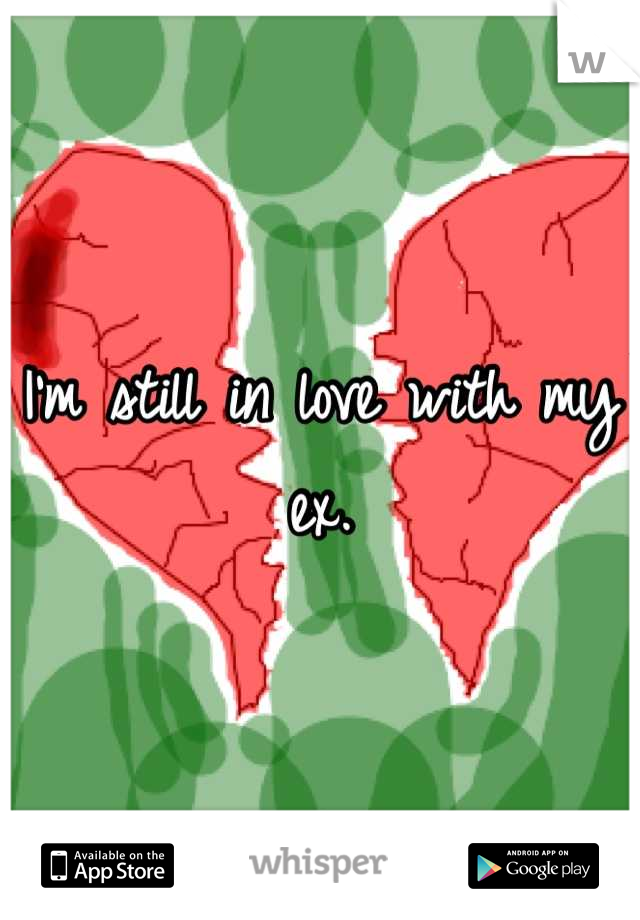The image is a detailed screenshot of an app advertisement, prominently featuring a broken pink heart split down the middle with the text, "I'm still in love with my ex," superimposed at the center. The heart is set against a patterned green background with varying shades of light and dark green. In the upper right corner of the image is a "W" logo, partially folded, indicating the app's branding. At the bottom, the ad highlights its availability on multiple platforms with two black rectangles: the left one saying, "Available on the App Store" accompanied by an iPhone logo, and the right one stating, "Android app on Google Play." Centered between these rectangles is the app's name, "Whisper," written in grey font.